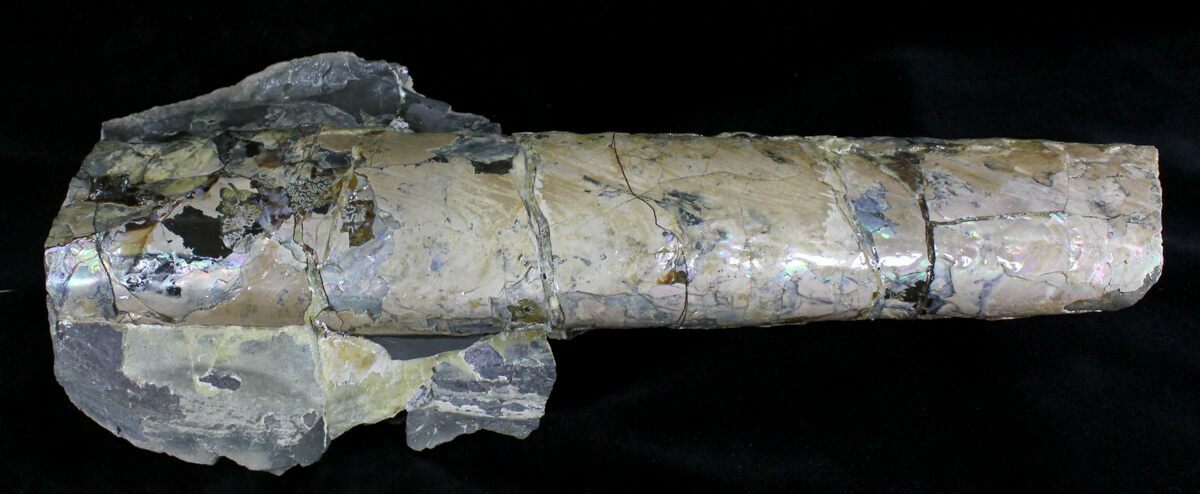The photograph captures a worn, rectangular stone object, laying horizontally against a pure black background. The stone, modeled in a blend of beige and gray, prominently features a mother of pearl sheen along the left and right bottom portions. Its surface is crisscrossed with various cracks: a black crack on the right side, followed by a beige crack to its left, a black hairline crack next, and a greenish gray crack further left. The left side of the object appears significantly damaged, marked by black, green, and white spots. Above and below this left portion, there's a rocky-looking mound, dark gray on top and a mix of dark gray and olive green at the bottom, giving a textured, layered appearance. The stone's overall coloration incorporates pearlescent tones, whitish blue hues, tan areas, and dark spots, adding to its ancient, relic-like aura.